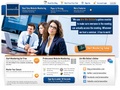This image features a screenshot of a professional networking website, likely LinkedIn, though the poor resolution and small size make it challenging to confirm. It displays a typical layout, starting with a rectangular blue banner at the very top, housing white text options that are indistinguishable due to blurriness. Above this blue banner, there are more sections of smaller text that might include navigational options like 'Services' or 'Blog.'

The central portion of the screenshot is dominated by an image of three individuals dressed in business attire. They are seated at what appears to be a conference table or desk. Two of the people are intently looking at a laptop, while the third person is looking directly at the viewer, engaging eye contact. Surrounding this image, there are various sections of text; most of the text is white, but some portions are highlighted or colored golden, possibly emphasizing quotes or important information. 

Adjacent to the image is a noticeable yellow rectangular shape that resembles a clickable button, although the blurriness makes it unclear whether it is an actionable element or simply highlighted text. Below this photo are additional lines of text and a box to input information, which could be a search field or a sign-up form for a newsletter. Further down, visible underlined links suggest additional clickable options, but the text is too illegible to read or interpret fully.

Overall, the layout and visual elements indicate a structured, professional website, mirroring the design sensibilities of LinkedIn or similar platforms.